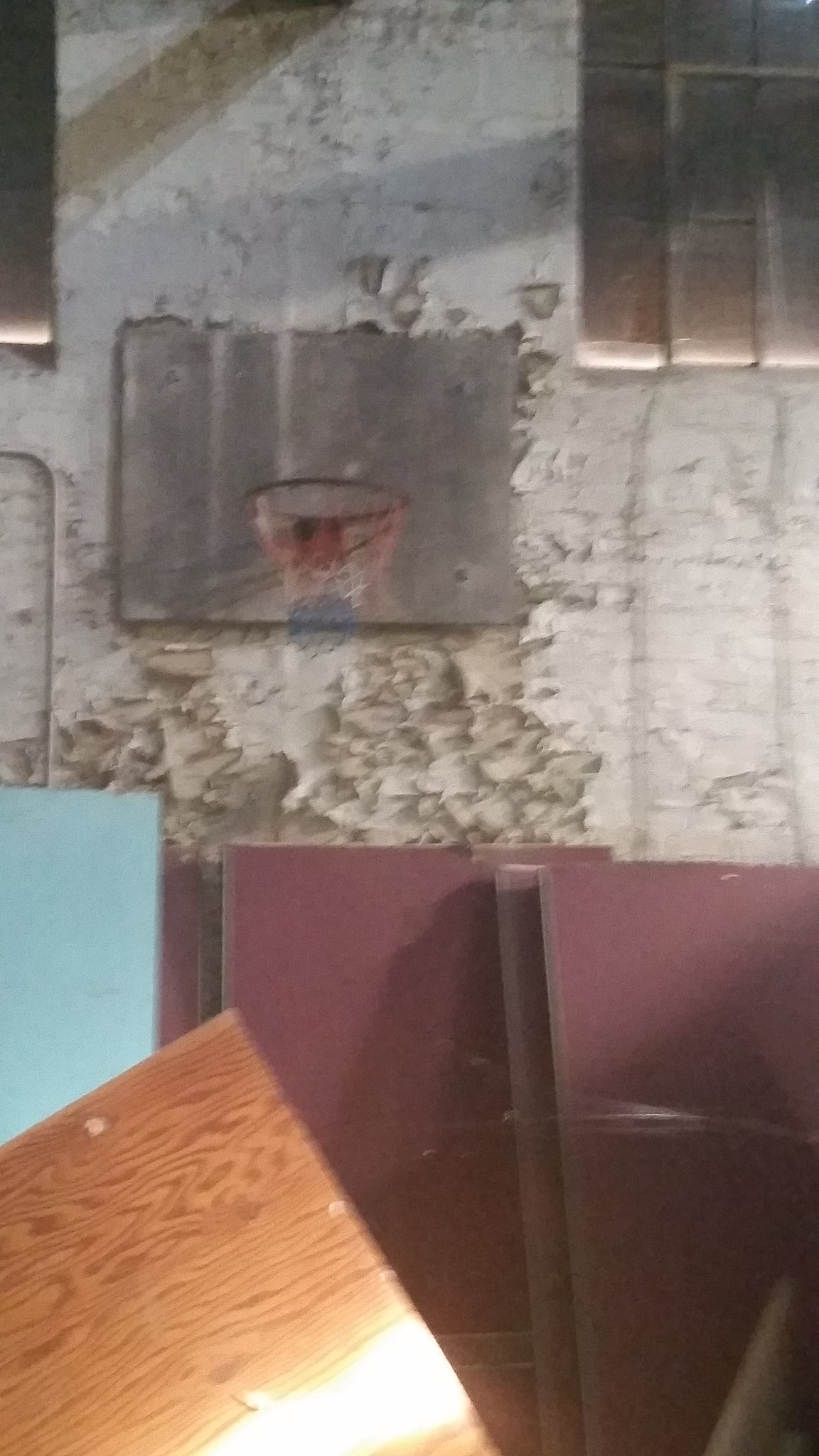The image captures a portrait-style photograph of a weathered, abandoned-looking building wall. The wall is painted white, but the paint is peeling off to reveal the gray brick underneath, giving it a dilapidated appearance. The focal point of the image is an old basketball hoop with a net colored red at the top, white in the middle, and blue at the bottom, resembling the American flag. This hoop is mounted on a faded, gray, wooden backboard, which is affixed to the wall between two partially visible windows with black bars. Below the hoop, various pieces of lumber and flat boards are leaning against the building. These include vertical boards in different colors—light blue, maroon, brown, and dark red. The scene is illuminated by sunlight, emphasizing the textures and colors, and adding a further sense of decay and abandonment to the setting.